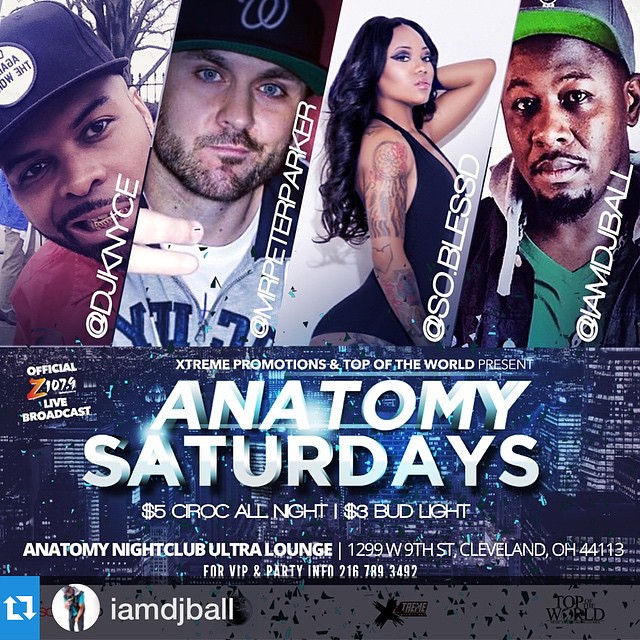The flyer is an advertisement for an event titled "Anatomy Saturdays," presented by Extreme Promotions and Top of the World. The top section of the flyer showcases four performer photos, almost vertically aligned from left to right. The first image features DJ KNYCE, a black man with a gold grill and a hat, identified by the handle @djkncyce. Next is Mr. Peter Parker, a white man in a hat and jersey, with the handle @mpreperparker. Third, we see S.O. Blessed, a black woman with tattoos on her right arm, turned to the side in a black unitard, identified by the handle @s.o.blessd. Lastly, is I am DJ Ball, a black man in a green hat, with the handle @imdjball. 

Below the performer lineup, the event details are listed: "Anatomy Saturdays" followed by "$5 Ciroc All Night" and "$3 Bud Light." The venue is Anatomy Nightclub Ultra Lounge located at 1299 9th Street, Cleveland, Ohio 44113. For VIP and party information, attendees are encouraged to contact 216-789-3492. The bottom of the flyer features a circular profile picture of DJ Ball against a black speckled background, reiterating his name and handle, "I am DJ Ball."